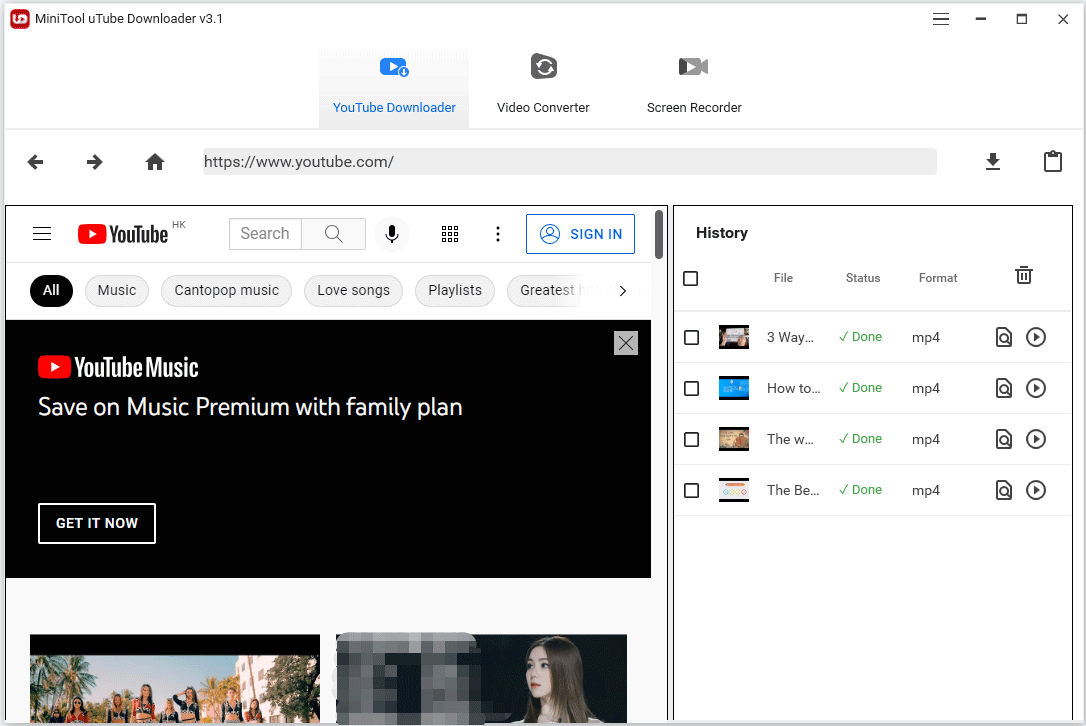The image depicts a bustling YouTube Music page, seemingly offering a mix of both free and premium services, possibly through YouTube Plus. The page layout is multi-columned but not overwhelmingly complex. On the left side, there's a navigation column with options such as the YouTube logo, a search bar, a sign-in button, and a speaker icon for voice search functionality. Below these options are categories like "Music," "Canton Pop Music," "Love Songs," and "Playlists," accompanied by an arrow indicating further listening options.

Central to the page is a prominent black banner advertising YouTube Music Premium. The banner highlights cost-saving opportunities with a family plan, and includes a "Get it Now" button for immediate purchase, along with an 'X' for closing the ad. Below this banner are partially visible, random images, perhaps thumbnails or album covers, which are difficult to discern. Lastly, a history section chronicles the user’s listening activity in a visually cluttered format.